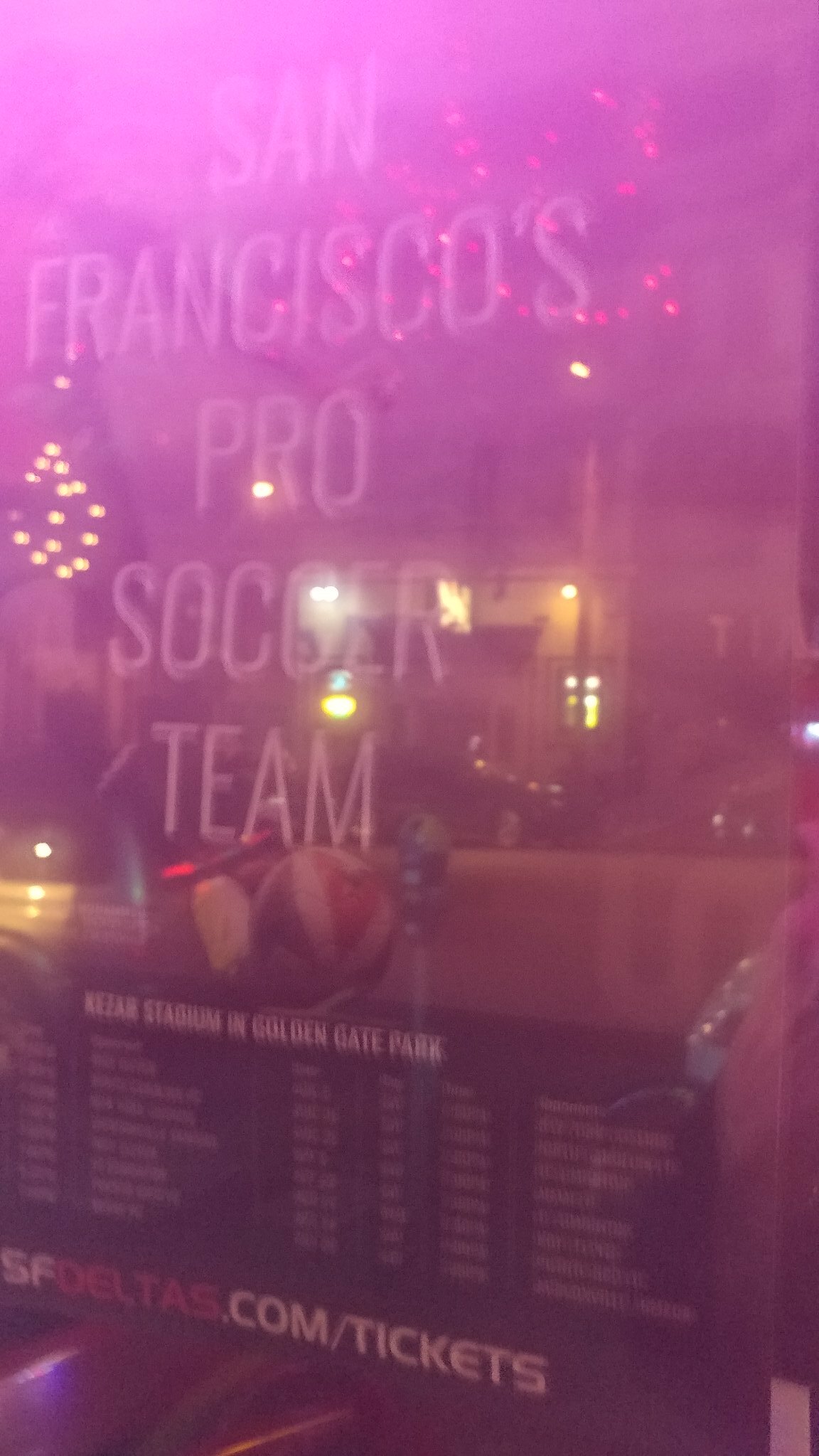This image is a low-resolution, somewhat blurry photograph of a business window in San Francisco, reflecting an overall purplish hue. Behind the glass, a neon sign announces "San Francisco's Pro Soccer Team," though the white neon lights appear turned off. Directly below, a black banner displays the URL "sfdeltas.com/tickets," with the word "deltas" highlighted in red, and a smaller list of text beneath that. Partially visible in the center is an image resembling a volleyball. Additional elements include a gray parking meter on the right and a black football on the left. In the background, there is a faint reflection of a building with some lit windows, suggesting it might be nighttime. The sign also mentions "Golden Gate Park," which adds context to the location. Overhead lights further obscure the details, adding to the image's unclear quality.